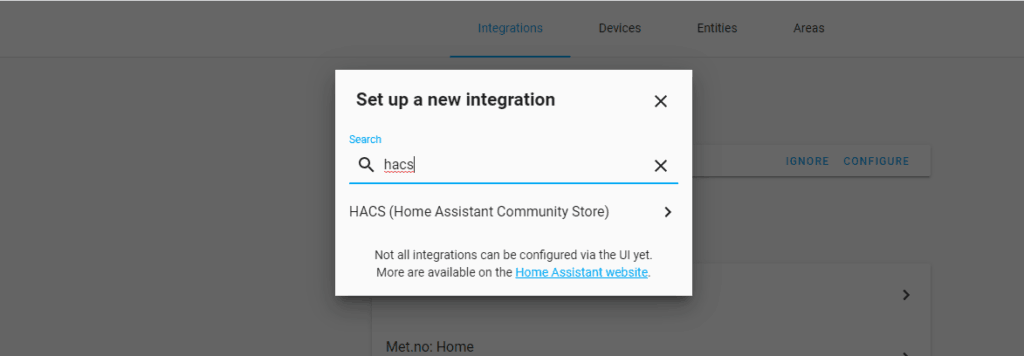The image is a screenshot of a web page focused on setting up a new integration within a software interface. The interface has a dark grayish filter overlay, and at the very top is a horizontal menu bar. The menu includes options labeled "Integrations," "Devices," "Entities," and "Areas," with "Integrations" currently selected, highlighted in blue, and underlined. The other menu items are displayed in dark gray.

Below the menu bar are two white interactive boxes. The first box has blue text with the options "Ignore" and "Configure." Further down at the bottom, another white box displays the text "met.no: home."

The main focal point of the screenshot is a large, horizontal white box centered at the top of the screen. This box is titled "Set up a new integration" in black text, and there is a small "X" icon on the right-hand side to close the box.

Directly below the title is the word "Search" in blue text, followed by a search bar containing a partial input "HACS" and a small search icon to the left. Below the search bar, the search result "HACS (Home Assistant Community Store)" is displayed, accompanied by a small arrow icon on the right. There is also a notice stating that not all integrations can be configured via the user interface yet, and more are available through the Home Assistant website, with the website linked in blue text.